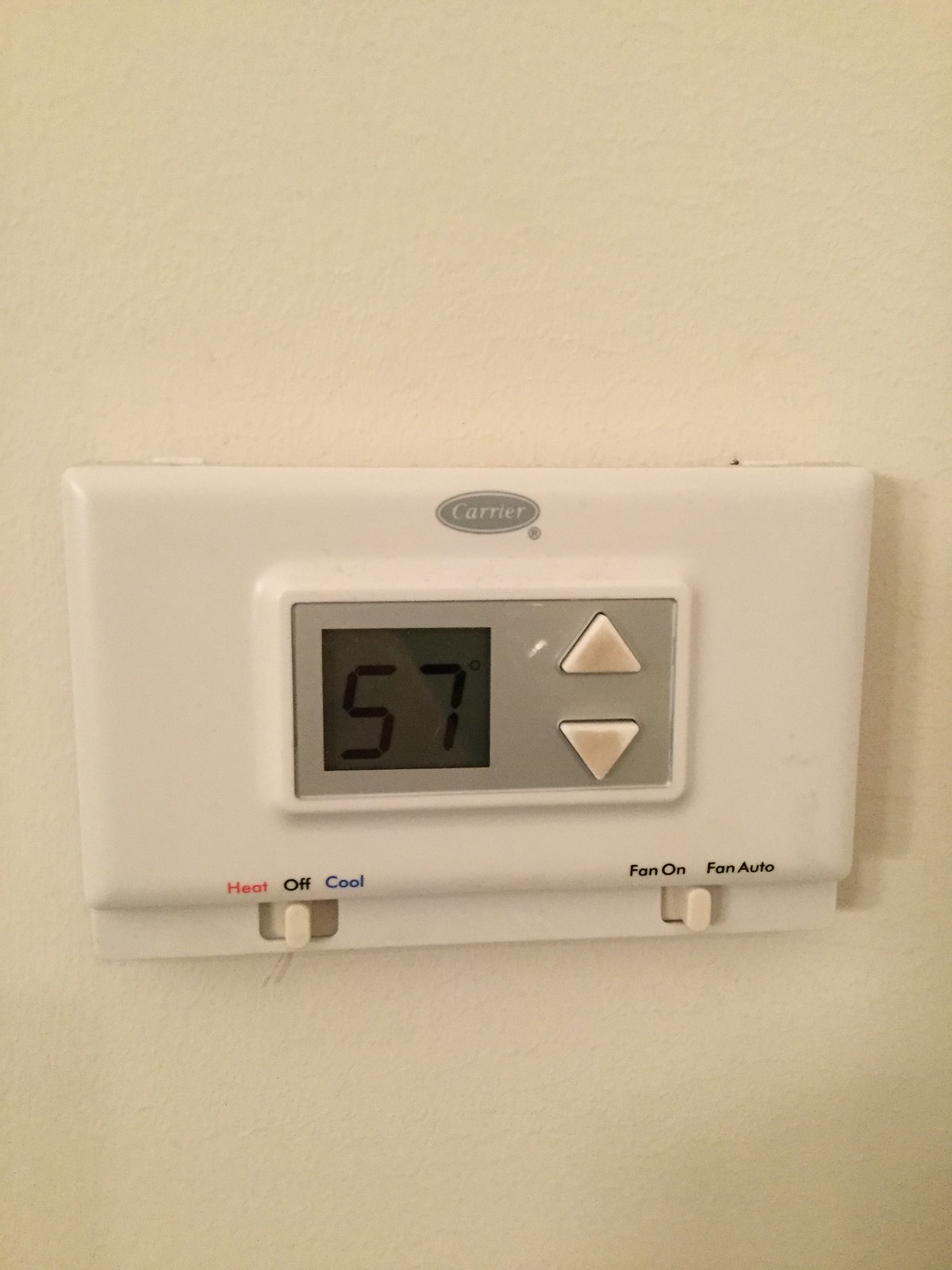This photograph captures a rectangular thermostat mounted on a wall, designed for a Carrier air conditioning and heating system. The digital display, set to "57" degrees, suggests the current room temperature. The thermostat features prominently used up and down arrows, indicating that the previous owner frequently adjusted the settings. It is currently in the "Off" mode, though it could be set to "Heat" (left) or "Cool" (right). Additionally, the options for "Fan On" and "Fan Auto" are visible, with "Fan Auto" being selected. The "Carrier" logo is prominently displayed at the top center of the thermostat, indicating the manufacturer's brand.